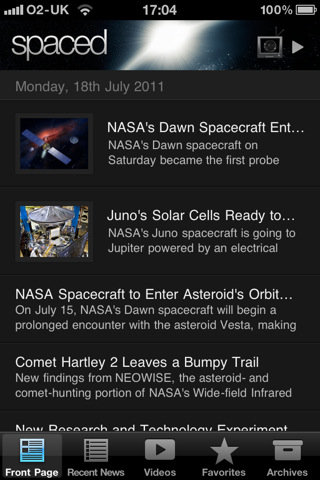### Detailed Caption for the Smartphone Screenshot

In this smartphone screenshot with a black background and white text, the screen is displaying a webpage. At the top of the screen, there is a status bar with several icons and numbers. From left to right, it includes:
- A Wi-Fi icon
- A battery icon showing 100% charge
- The text "02-UK"
- A Wi-Fi icon again 
- The time "17:04"
- Another battery icon showing full charge

Below the status bar, the screen is divided into several sections. The first section contains:
- An image of outer space, resembling the Sombrero Galaxy, positioned towards the right with a right-facing arrow next to it
- The day and date "Monday, 18th of July, 2011"

The next section displays:
- An image of a satellite in space, accompanied by text on its right side: "NASA's Dawn spacecraft", followed by an ellipsis. The subtitle reads: "NASA's Dawn spacecraft on Saturday became the first probe."

The subsequent section features:
- An image of another satellite, seemingly located in a warehouse or indoor setting, with text to its right: "Juno's solar cells ready to", followed by an ellipsis. The subtitle mentions: "NASA's Juno spacecraft is going to Jupiter, powered by an electrical" (the sentence cuts off here).

Further down the screen, there is additional text:
- "NASA's spacecraft into asteroid's orbit..." indicating an article or news snippet, and notes that "On July 15th, NASA's Dawn spacecraft will begin a prolonged encounter with the asteroid Vesta, making" (the text cuts off here).
- "Comet Harley 2 leaves a bumpy trail", with subtext: "new findings from neowise.org and the asteroid and comet hunting portion of NASA's Wide Field Infrared" (the sentence is cut off here).

At the bottom of the screen, there are tabs labeled:
- "Front Page" (the currently selected tab)
- "Recent News"
- "Videos"
- "Favorites"
- "Archives"

This detailed description captures all elements and text present in the smartphone screenshot, providing a clear and structured overview of the content displayed.